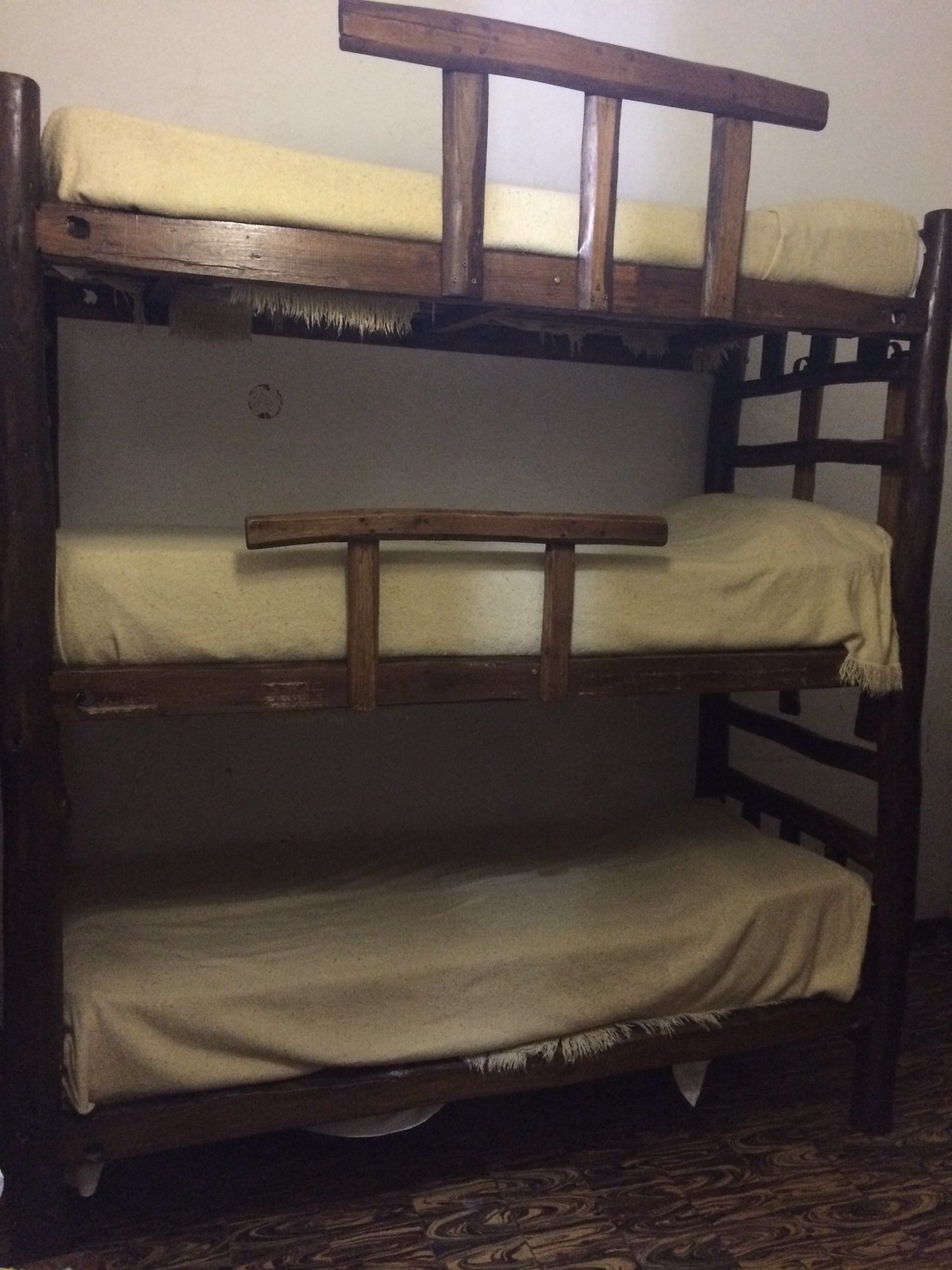The image depicts a rustic, wooden triple-decker bunk bed viewed from the right-hand side. Each of the three beds is neatly made with thin, tan blankets tucked tightly around white mattresses, featuring delicate ruffled edges. Each bunk is further equipped with a pillow, creating a uniform and ready-to-use appearance. The highest bed has a more prominent railing compared to the middle one, which has a lower guard rail. Instead of a conventional ladder, the bunks are accessed by rung-like structures on the side, though a proper ladder might be present out of the frame on the left-hand side. The setting suggests a hostel or a space-efficient accommodation, with the flooring featuring vintage brown and cream-colored, psychedelic-patterned carpet reminiscent of the 1970s. The overall photographic quality is not optimal, potentially due to poor lighting or camera, yet it distinctly captures the unique sleeping arrangement in this room.